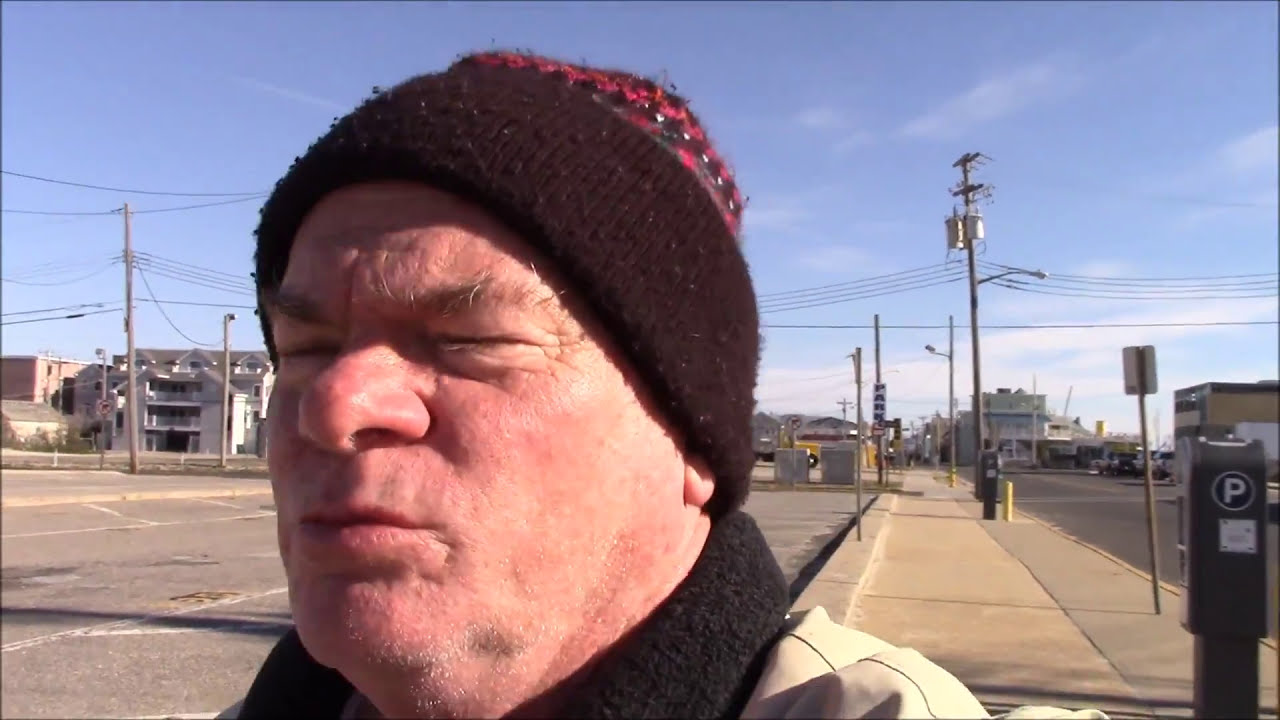In this image, an older man, possibly in his 50s or 60s, stands prominently in the center. He is looking off to the left with his eyes squinted or possibly closed, likely due to the sun shining on his face. The man is dressed for the cold weather, wearing a distinctive wool hat with a black brim and a fuzzy pattern of red, gray, and black on top. His black jacket features a tan body with a black, fleece-like collar. He has some scruff on his chin, visible amidst his white facial hair.

The scene is set outdoors on a desolate winter day, giving off a cold atmosphere. In the background, there is a sidewalk running behind the man, a payphone, and a few signs. To his left is a vast, empty parking lot with some cars and a parking meter visible. Various buildings are scattered in the distance, while numerous power lines and light poles crisscross the sky, which is dotted with light clouds. The overall tones of the image include shades of gray, yellow, pink, red, brown, black, blue, and light blue, all contributing to the chilly and somewhat bleak street setting.